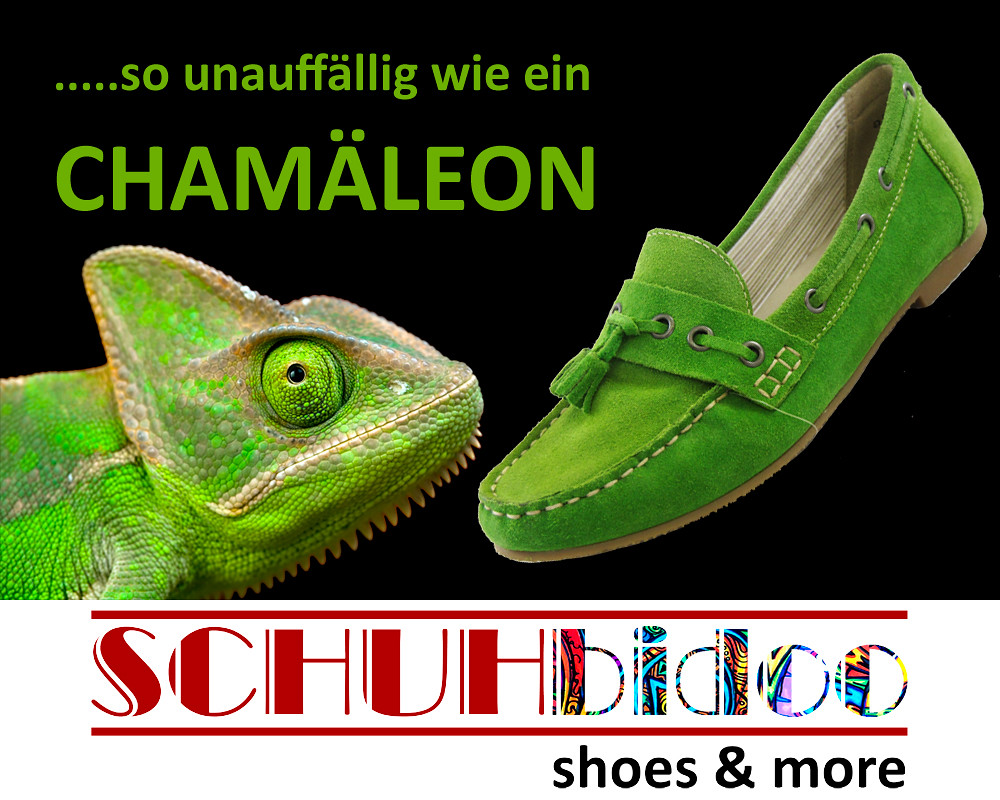The advertisement features a striking visual comparison between a bright green chameleon and a pair of moccasin-like shoes in the exact same shade of green. The background of the image is black, and the top section includes green text that appears to be in German or Swedish, with an excerpt mentioning a chameleon. On the left-hand side, there's a close-up of the chameleon's face, notable for its bright green color, horned head, and round eyes. Just beside the chameleon is the green moccasin, crafted from brushed bright green leather, featuring tan stitching, tan soles, white interior, silver eyelets, and a tassel on the front. The shoe's colors and texture mimic the chameleon's appearance. At the bottom of the advertisement, the brand "Shabby-Doo" is displayed, with 'Shuh' in a bold red font and 'Bidoo' in a multicolored, animal print-inspired font. Beneath this logo, the text reads "Shoes and More."